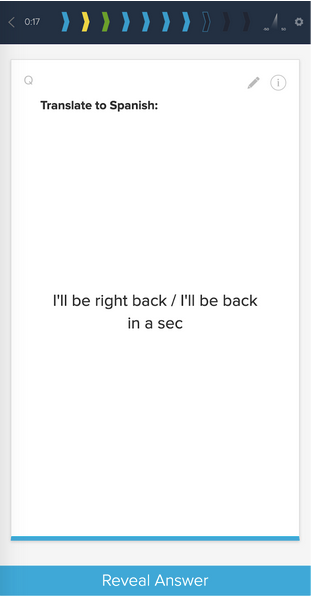The image appears to be a screenshot from a language translation teaching program. At the very top of the interface, there are various colored elements and a timestamp reading "0.017". An arrow pointing upwards suggests a back navigation option, and the background of the top banner is dark. To the right is a cog icon indicating access to settings. 

On the top left, there is a white blank sheet next to a "Q" icon. Below that, a bold statement declares "Translate to Spanish". Also visible are a pencil icon and an eye icon encircled, likely for editing and preview functions, respectively. 

In the middle of the screenshot, black text displays the phrase "I'll be right back / I'll be back in a sec." At the very bottom, there is a prominent blue button labeled "Reveal Answer" in white text. All the elements are distinct and separated from one another, making the interface clean and organized.